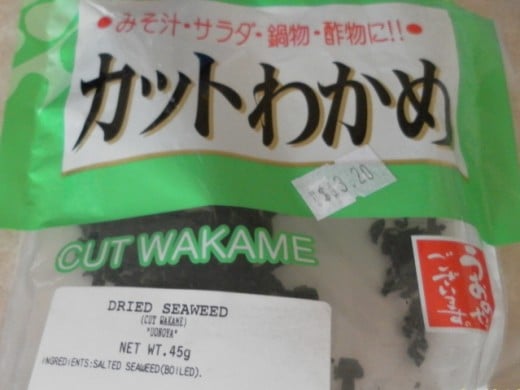This image features a package of dried seaweed that occupies the entire frame. The upper section of the package has a prominent white rectangle containing text in another language, likely Chinese or Japanese, with red characters at the top and larger black characters underneath. Below this text block is a small white price tag displaying $13.20. The upper background of the package is bright green, transitioning into a see-through section in the lower part, revealing dark forest green seaweed inside.

Centrally positioned on the package, “Cut Wakame” is written in white, outlined with green. In the bottom left corner, a larger rectangular label provides additional details: “Dried Seaweed” in black text, followed by “Net Weight 0.45 grams.” The ingredients list includes “Salted Seaweed” with “boiled” in parentheses. A small red sticker is also visible on the right side of the packaging.